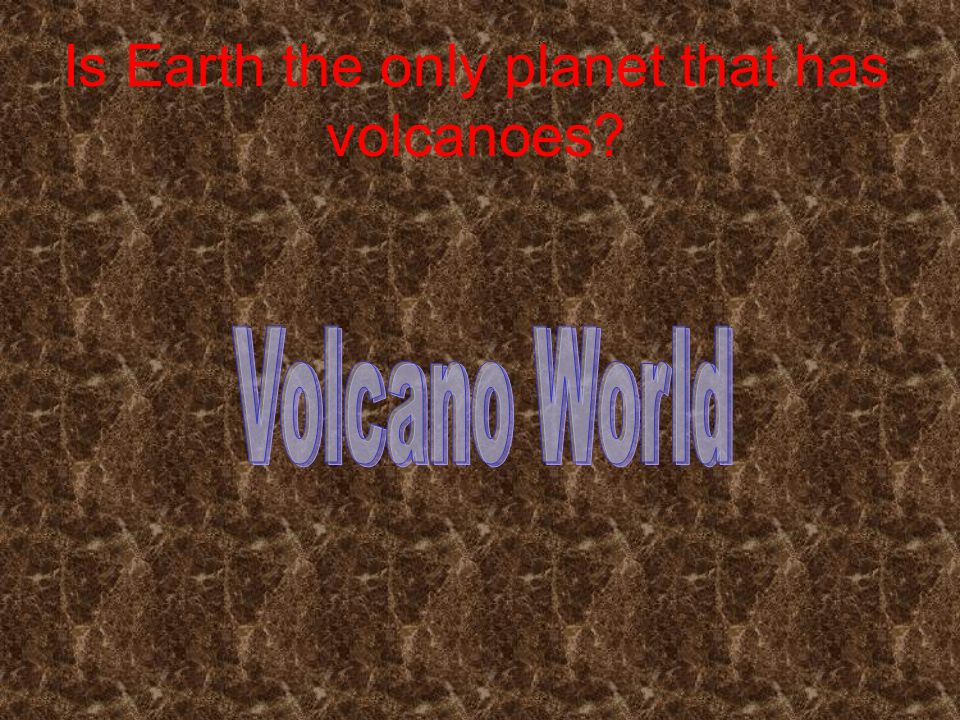The image features a textured brown background, resembling leather and varying from dark brown to light tan. The pattern, suggestive of the Grand Knight's move zigzagging symmetrically, appears abstract yet repetitive, and upon close inspection, one might even perceive a resemblance to a person's likeness, such as LeBron James, integrated into the design. At the top, there is a striking red, sans serif font asking, "Is Earth the only planet that has volcanoes?" In the center, in a bold, light purple font with a shadow effect, are the capitalized words "Volcano World." This text is neatly embedded in the intricate background and is the only text within the image, suggesting it could be from a textbook or an article.